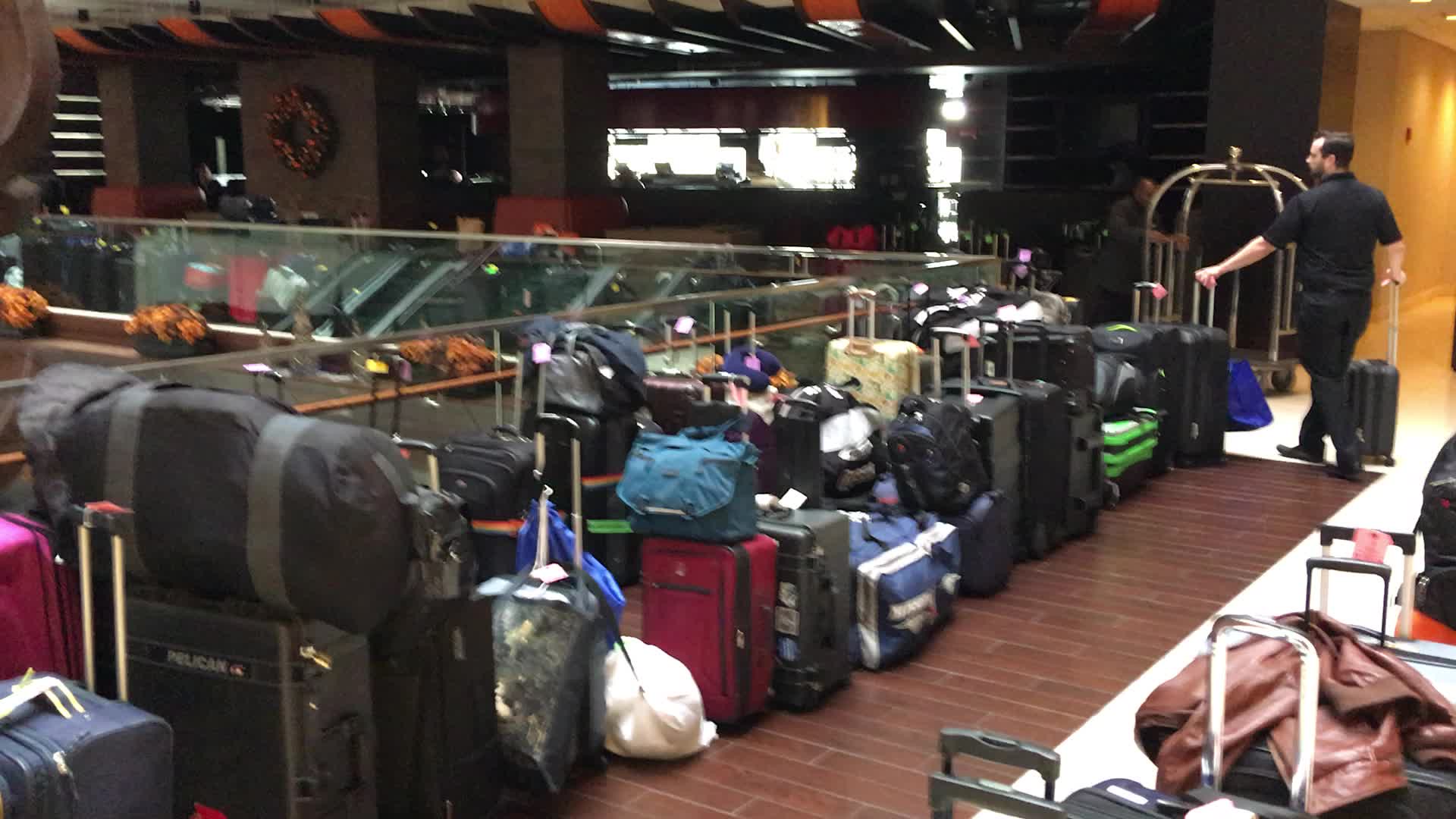The image captures a bustling hotel lobby filled with a diverse array of luggage of various sizes, colors, and types including red and blue suitcases, duffel bags, backpacks, and carry-on bags. The luggage is densely packed and positioned both in front of a glass railing and in the bottom right corner on different floorings – brick tiles and a white surface. A man with brown hair, dressed in a black short-sleeve polo shirt, black pants, and sneakers is the focal point. He appears to be a hotel staff member, handling two black suitcases. In the background, a second man in a long-sleeve black shirt is seen pulling a gold-colored luggage rack. The scene includes additional details such as an escalator and windows in the upper portion of the image, orange flowers evenly spaced along the railing near the escalator, and a brown column adorned with a Christmas wreath.